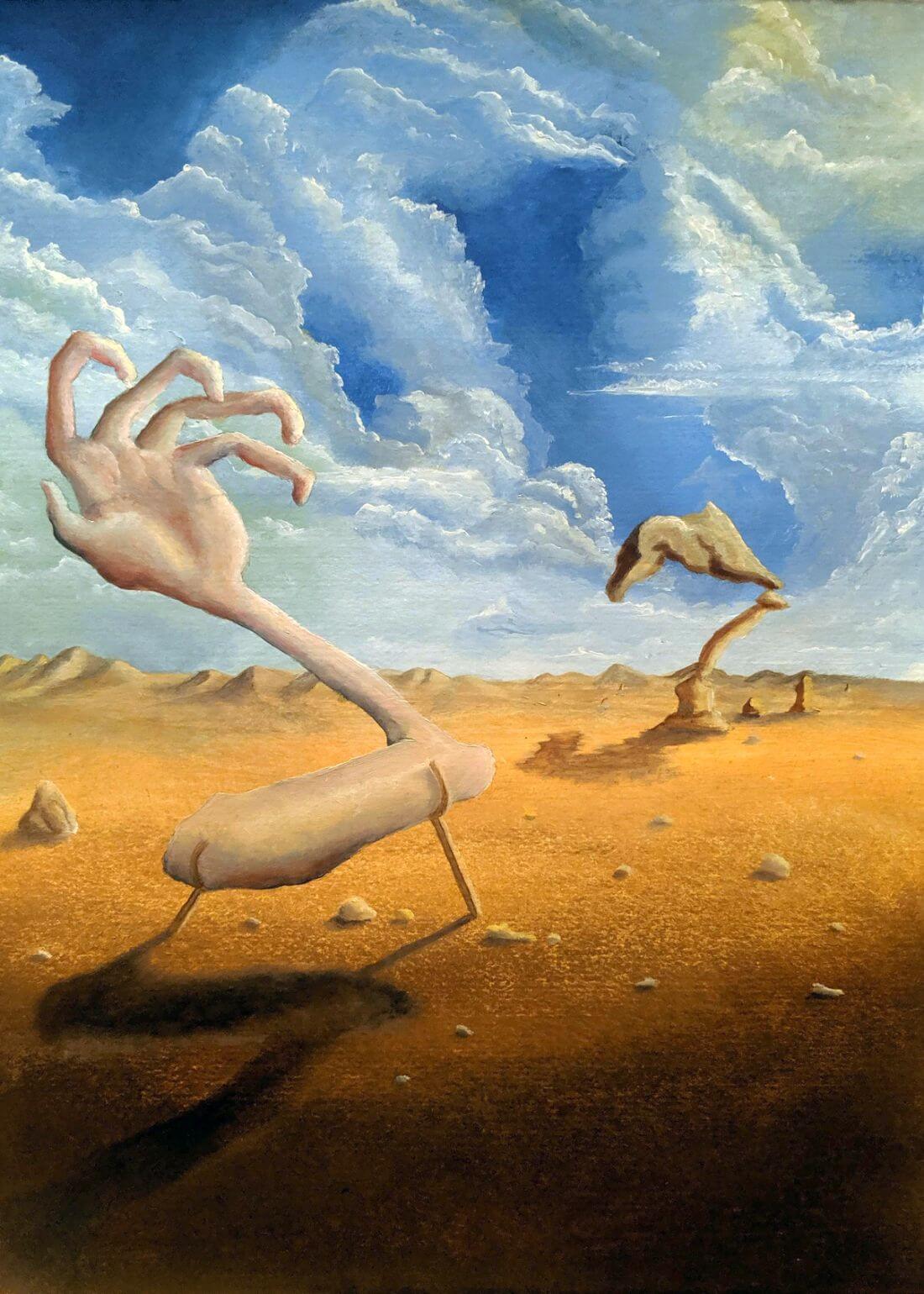This surrealistic painting, reminiscent of Salvador Dali's style, depicts a barren desert landscape under a partly cloudy sky with subtle sunlight peeking from the upper right corner. Central to the image is an oversized, disembodied arm resembling a giant's limb, severed at the shoulder and awkwardly propped up by two wooden stakes. The arm's hand rests palm-up, its fingers deformed into a claw-like shape, towards the upper part of the image. To the left, a second white hand-like structure appears, its fingers curling inward, adding to the otherworldly ambiance. In the background, rock formations and curious shapes—one notably resembling the head of a dinosaur or duck—jut out from the desert sands. The ground is depicted with shades of dark brown and tan, featuring scattered rocks and sand dunes, enhancing the post-apocalyptic aura. Various elements, including the sky with its puffy white clouds and the desolate terrain, are rendered in a distinctly surrealistic, dream-like fashion, true to Dali's artistic influence.